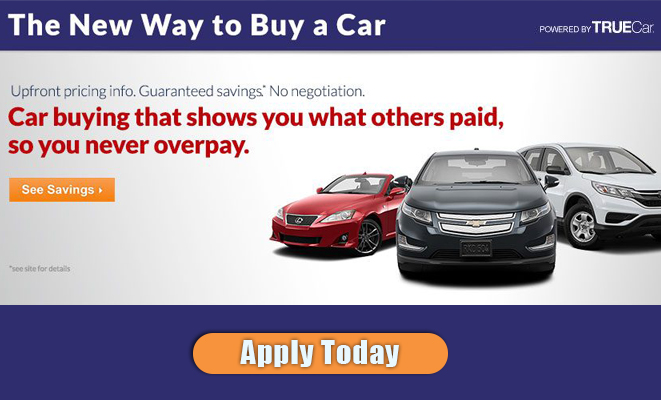The image appears to be an advertisement for a service called "Powered by Truecar". 

At the top, there's a blue banner featuring bold white text on the left side that reads, "A new way to buy a car." On the right side of the banner, in smaller white letters, it states, "Powered by Truecar".

Below the blue banner, the background transitions to white. In this section, there are several lines of text. In gray letters, it lists "upfront pricing information," "guaranteed savings," and "no negotiation." Following this, in red letters, it reads, "Car buying that shows you what others pay so you never overpay."

Beneath the text, there's an orange rectangular button with the phrase "See Savings" written in white letters. 

The next part of the image displays pictures of three different vehicles: a red convertible of an unspecified make, a gray Chevrolet car, and a white SUV.

Below the vehicle images, there's another blue banner. This one features an orange, pill-shaped button with white text that says, "Apply Today".

This ad seems to promote a car-buying website where users can research vehicles, see potential savings, and apply for purchasing.